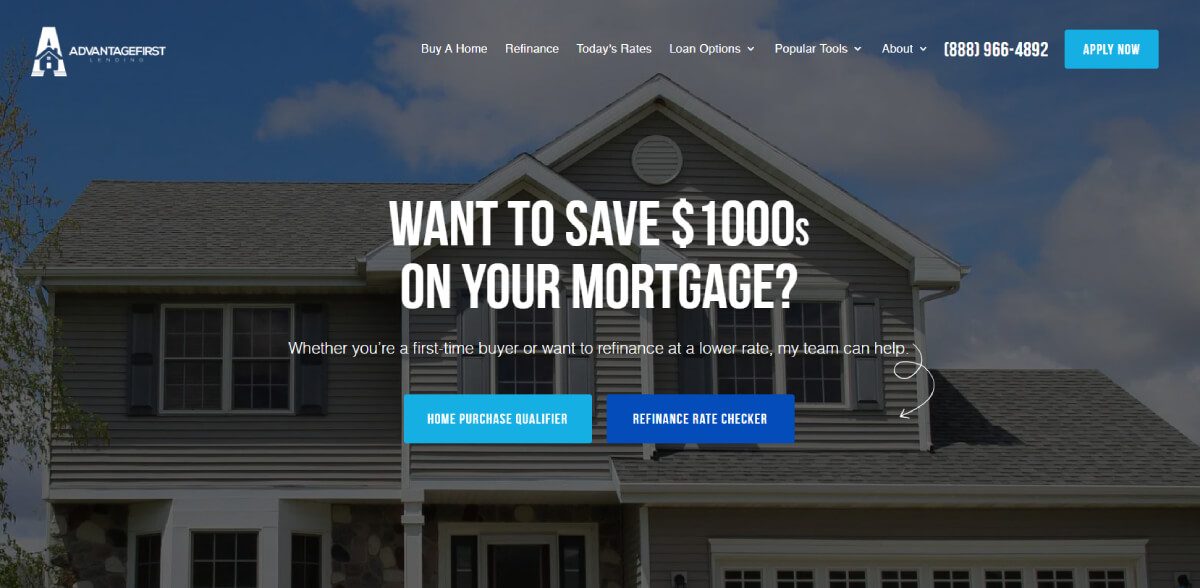### Caption:

This is a screenshot of a website header, displayed in a wide landscape format. In the top left corner, the header features the brand's logo: a stylized "A" incorporating a house symbol. Next to the logo text, "Advantage First," is a small, almost unreadable slogan due to the image size.

To the right of the logo, the navigation menu begins, spanning the remainder of the header. The items are in white title-case text and include:
- Buy a Home
- Refinance
- Today's Rate
- Loan Options (drop-down menu)
- Popular Tools (drop-down menu)
- About (drop-down menu)

Further right, there's a bold white phone number: "(888) 966-4892." Next to the phone number, a light blue button with rounded corners features the text "Apply Now."

Centered below the navigation menu, a large heading reads: "Want to save thousands on your mortgage?" followed by a subheading: "Whether you're a first-time buyer or want to refinance at a lower rate, my team can help."

Underneath the subheading, two buttons are displayed:
- A light blue button labeled "Home Purchase Qualifier"
- A dark blue button labeled "Refinance Rate Checker"

The background image shows the top floor of a typical modern two-story house under a blue sky with fluffy white clouds. The image has a dark overlay to enhance text readability. A tree partially enters the view from the left side, adding a touch of natural element to the scene.